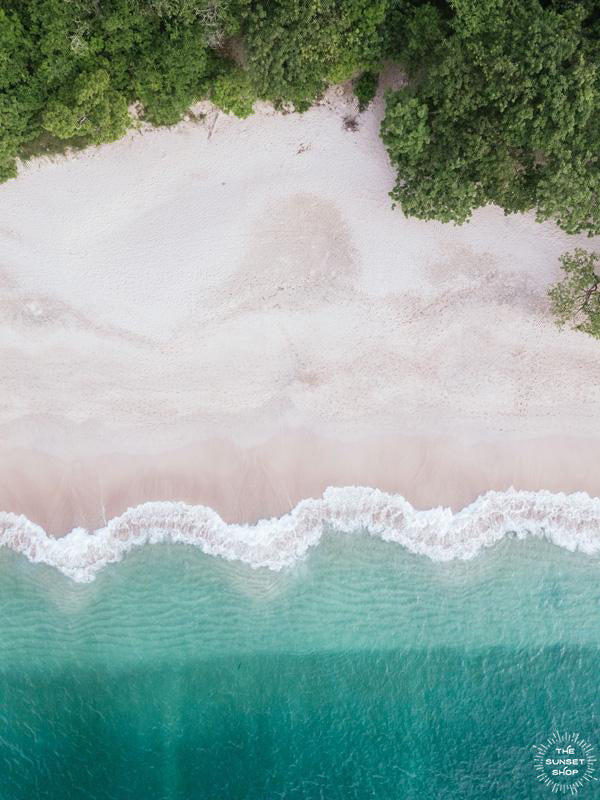This aerial photo captures a stunning tropical coastline, featuring a dynamic interplay of colors and textures. The lower portion of the image showcases a dark to light turquoise body of water, indicative of shallow tropical waters abruptly giving way to deeper, darker waters. Waves crash uniformly along the shoreline, forming a series of consistent arch shapes and creating a wavy white line where they meet the tan, sandy beach. The sand exhibits a mix of lighter and darker patches, some areas glistening as waves repeatedly rush in and recede. Towards the top of the image, lush greenery – likely a combination of trees and bushes – forms a vibrant tree line that spans from the left to the right, becoming denser towards the right side. In the bottom right corner, the image features a logo reading "The Sunset Shop" in white text, encircled by a design reminiscent of a sun with streaming rays.